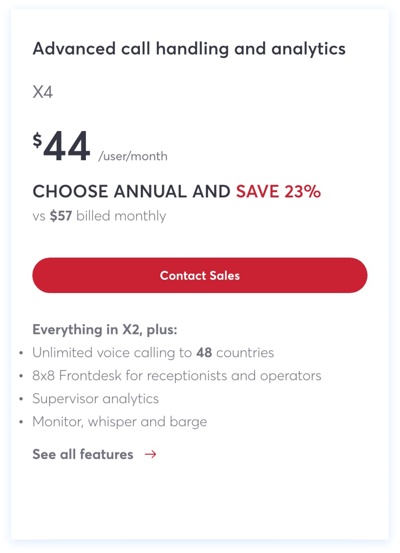This image features a screenshot set against a white background with a light gray border. At the top, bold black text reads "Advanced Call Handling and Analytics." Directly beneath that, "X4" is also displayed in bold black letters. Following that, the price "$44/user/month" is prominently shown, with a note reading "Choose annual and save 23% vs $57 billed monthly" just below it. Toward the bottom, a prominent red action button labeled "Contact Sales" is visible.

Further down, in an "Everything in x2 plus" section, several bullet points in clear text detail the additional features included. These features are as follows:

- Unlimited voice calling to 48 countries
- 8x8 front desk services for receptionists and operators
- Supervisor analytics
- Monitor, whisper, and barge functions

At the very bottom of the image, bold black text states "See all features," accompanied by a red arrow pointing to the right, which likely indicates further details available through a clickable link.